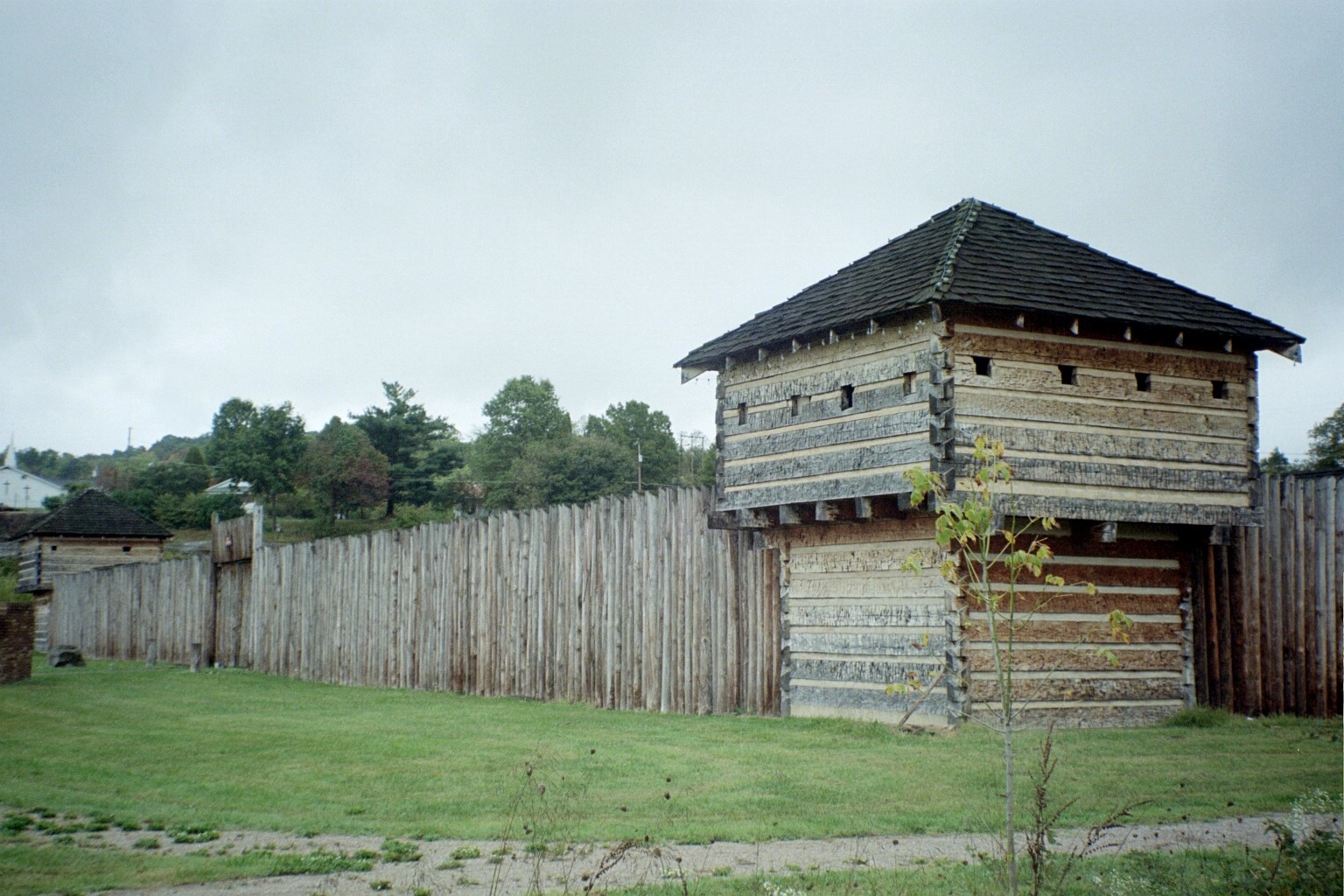The image showcases an outdoor scene with an old, small building that looks like two houses stacked on top of each other, featuring stone walls and a triangular roof with black shingles. This building has horizontal wooden slats on its lower portion and small, square cutout windows on the second floor. Surrounding this structure is a tall, weathered wooden fence made of vertical, worn, whitish-brown branches that stretches across most of the image. In the foreground, there’s a light brown dirt or gravel path running horizontally, flanked by short green grass and small trees or twigs. Tall green trees dominate the horizon on the left side of the photograph, while the upper portion of the image features a light gray sky with scattered white-gray clouds, adding to the antiquated atmosphere of the setting.